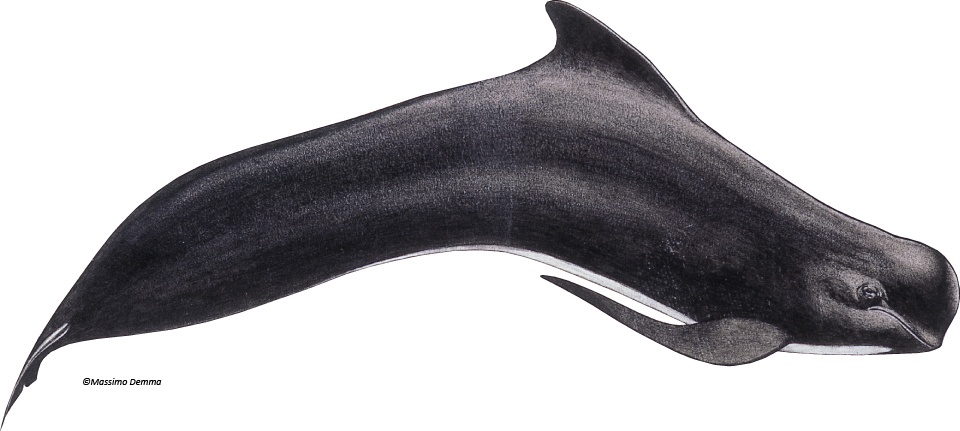Against a stark white background, there is a detailed drawing of a whale-like sea creature. The body curves upward at the midsection, enhancing its sleek, elongated appearance. This creature has a rounded head with a small, black eye and a downturned mouth, emphasizing a gentle, non-aggressive look. Though the jaw isn't pronounced, it seamlessly merges into a long, streamlined body devoid of a visible neck. A prominent dorsal fin sits atop its back, while a similarly shaped, flat-topped fin extends from the bottom. The creature's black body is contrasted by a strip of white running along the underside, implying a distinct underbelly. The tail fin is pointing straight downwards, obscuring any details of the rear side fins. At the bottom corner of the image, the text "Copyright M.A.S.S.I.M.O. D.E.M.M.A." is visible in black, hinting at the artwork's attribution. The image conveys the essence of a beluga whale, characterized by its rounded features and monochromatic color scheme, unified by the clean, white backdrop.